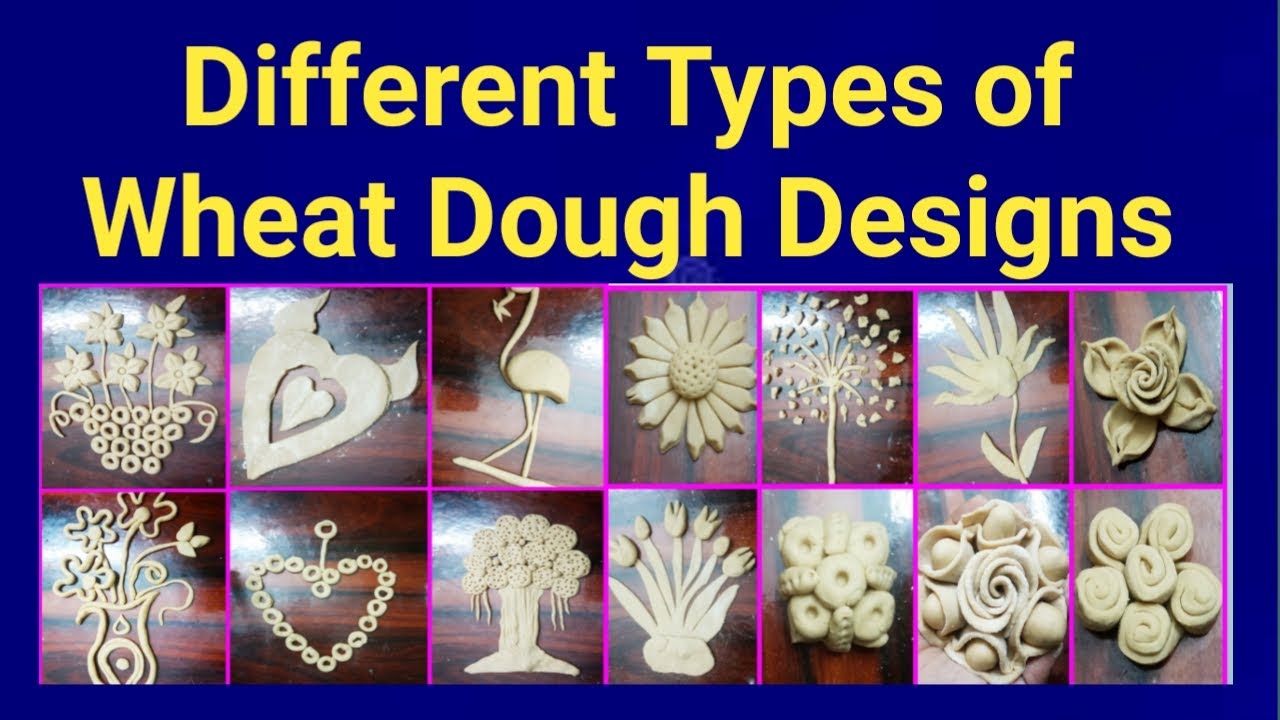The image is a dark navy blue rectangular infographic with bold yellow text at the top that reads "Different Types of Wheat Dough Designs." Below the title, there are two rows and seven columns of pictures, each bordered by a bright purple trim, showcasing various intricate wheat dough designs placed on a wooden surface. 

In the first row from left to right:
1. A vase or plant pot with flowers.
2. A heart with a smaller heart inside, adorned with what looks like devil horns or wings.
3. A flamingo.
4. A daisy.
5. A tree with leaves.
6. Another flower featuring longer petals.
7. A rose with leaves.

In the second row from left to right:
1. A vase or plant pot containing daisies.
2. A heart made out of circles, featuring a string and a small hook at the top.
3. A different type of tree with circular leaves and hanging branches, supported by a thick trunk.
4. An arrangement of tulips.
5. A cluster of circular flowers with chunky leaves interspersed.
6. A bouquet with roses and other floral elements.
7. A flower resembling the swirl of a cinnamon roll.